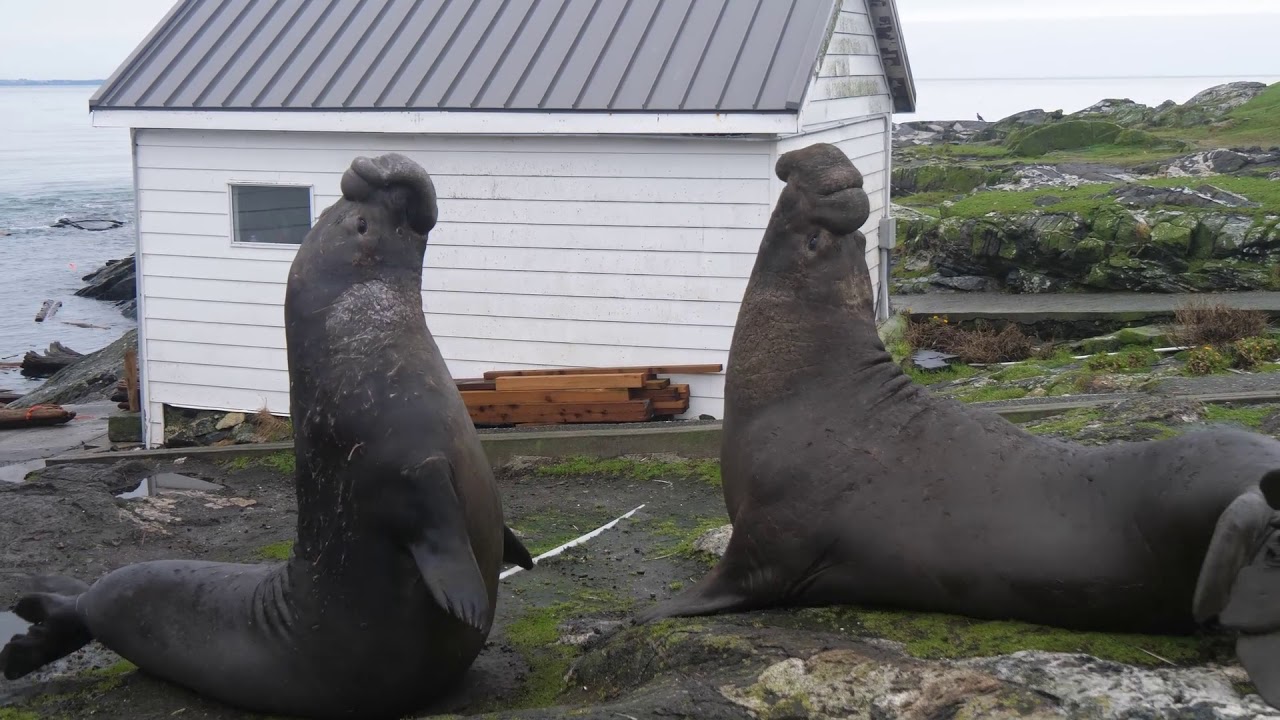This is a detailed color photograph capturing two lifelike sculptures of walruses, though they are sometimes mistaken for seals, positioned on a wet, rocky beach with patchy grass and moss. The walruses are facing each other, heads raised, with the one on the left having its flippers up and the one on the right resting its flippers on the ground. Between them is a gap of approximately two feet. In the background stands a small, white clapboard cottage with a gray wooden roof and a small window, along with some plywood and lumber stacked against it. Beyond the cottage, the sea is visible with rocky surfaces extending into the water, under a gray cloudy sky. There is an isolated patch of sandy beach amidst the rocky terrain. The scene is devoid of people, live animals, or vehicles, emphasizing the natural and serene coastal environment.